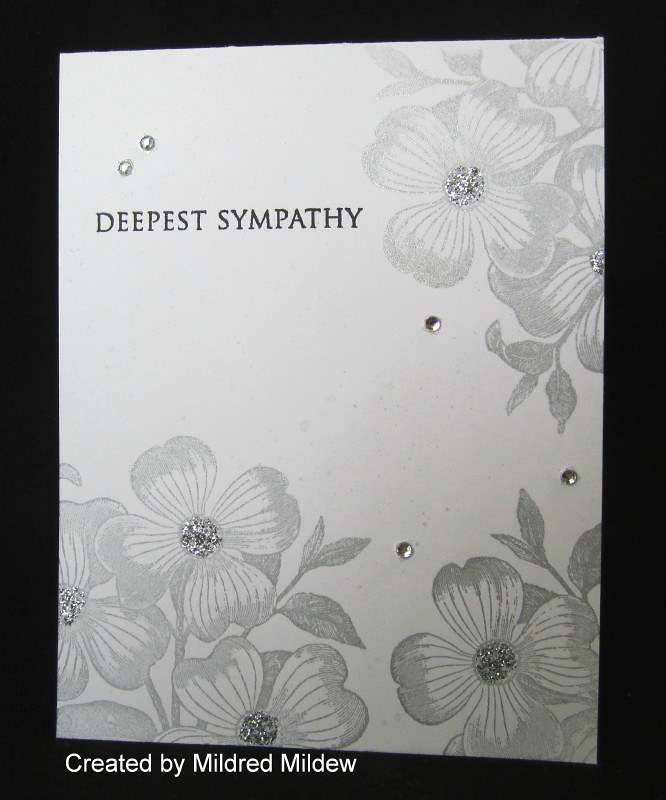The image showcases a tall, rectangular Sympathy card placed on a light gray piece of paper, all set against a completely black background. The card tilts slightly downward at the bottom right corner, creating a subtle dynamic effect. Prominently, in the upper left corner, the card reads "DEEPEST SYMPATHY" in bold, all-capital letters, with two rhinestones accentuating the double E's in "Deepest." The card is adorned with delicately pencil-colored floral motifs at the bottom left corner, upper right corner, and lower right corner. Each flower features heart-shaped leaves that darken towards the top, with a silver glitter circle at the center, adding a touch of sparkle. Additionally, small jewels are taped sporadically across the card, enhancing its intricate design. Below the card, against the black surface, is a white text that states, "CREATED BY MILDRED MILDEW," adding a personalized touch to this solemn and elegantly designed card.